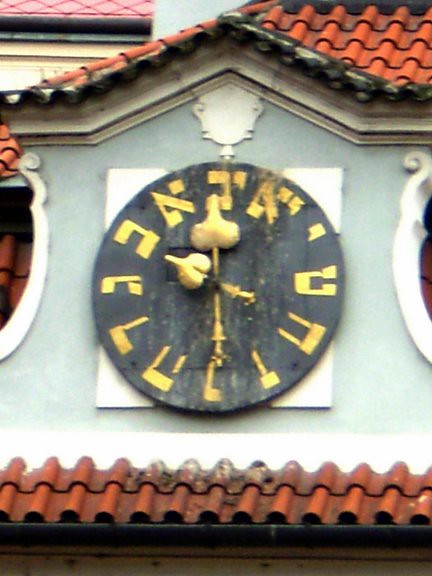This detailed photograph captures the upper section of a uniquely colored building. The structure is painted in a distinctive seafoam grayish hue that contrasts elegantly with its striking roof. The roof, primarily orange with black trimming, features a textured, bumpy surface and an arch-like design at its apex. 

Centrally positioned on the roof is a black, round clock, notable for its use of Hebrew letters in place of traditional numbers. This clock, adorned with gold hands and letters, rests on a white square backdrop. The Hebrew letters exhibit signs of aging, their golden paint slightly worn and weathered by time.

Flanking the clock, partially visible at the edges of the photograph, are two windows, further emphasizing the realism of this architectural scene. The overall style of the image is highly realistic, presenting a vivid portrayal of what appears to be a genuine location.